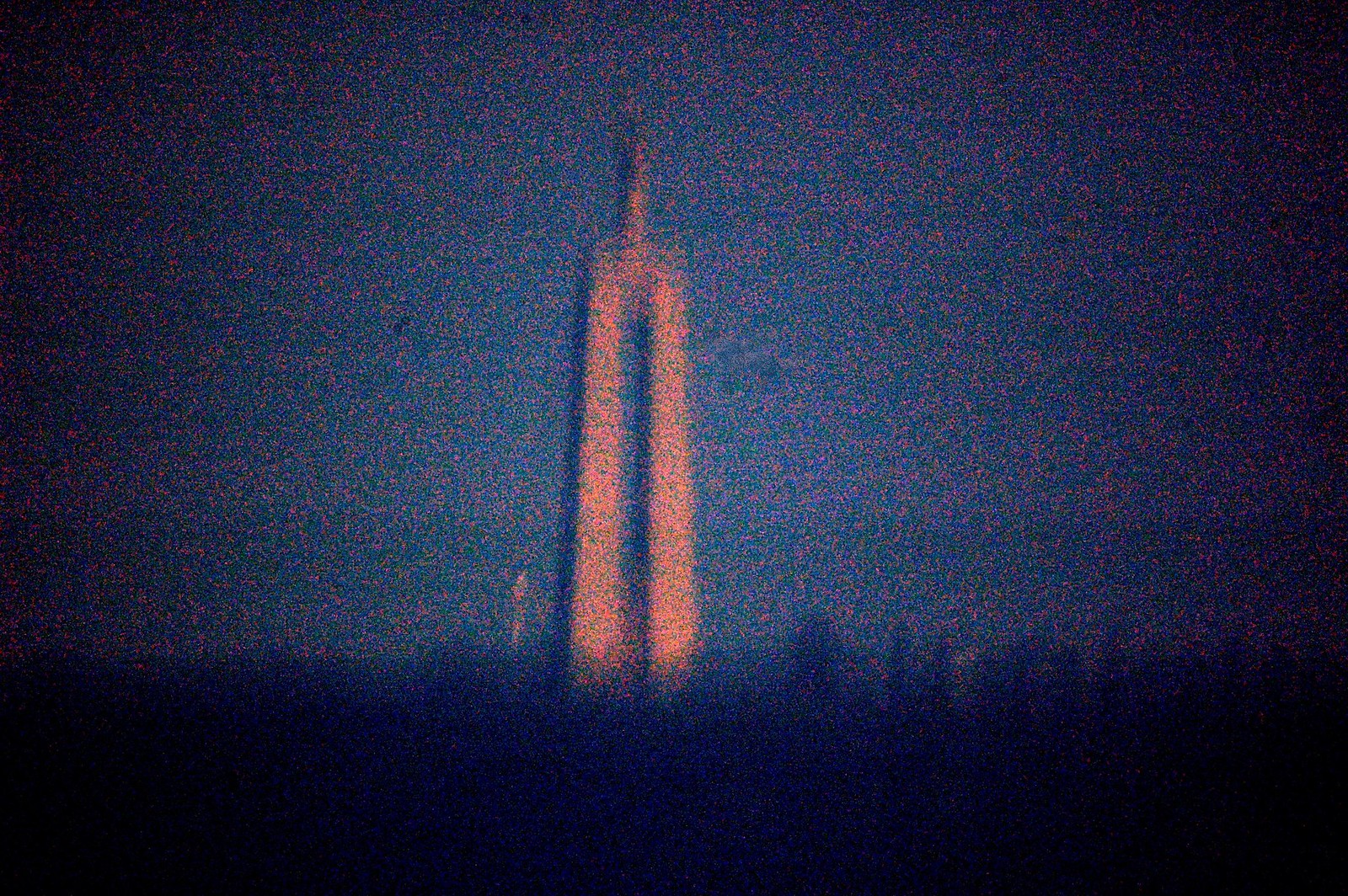The image is a low-quality, blurry photograph featuring a peculiar, large structure set against a purplish-blue background. The structure, which dominates the center of the image, appears to be fork-shaped with two prominent white lines running vertically and a connecting white line at the top, dividing it into sections. Below the structure, dark trees are visible in the bottom right corner. The photo seems to capture a time perhaps during sunrise or sunset, inferred from the soft, reflective light adding a subtle glow to the structure. Despite the heavy pixelation and blur, the image conveys a somewhat artistic, dreamlike quality, likely due to filters or the camera's settings.